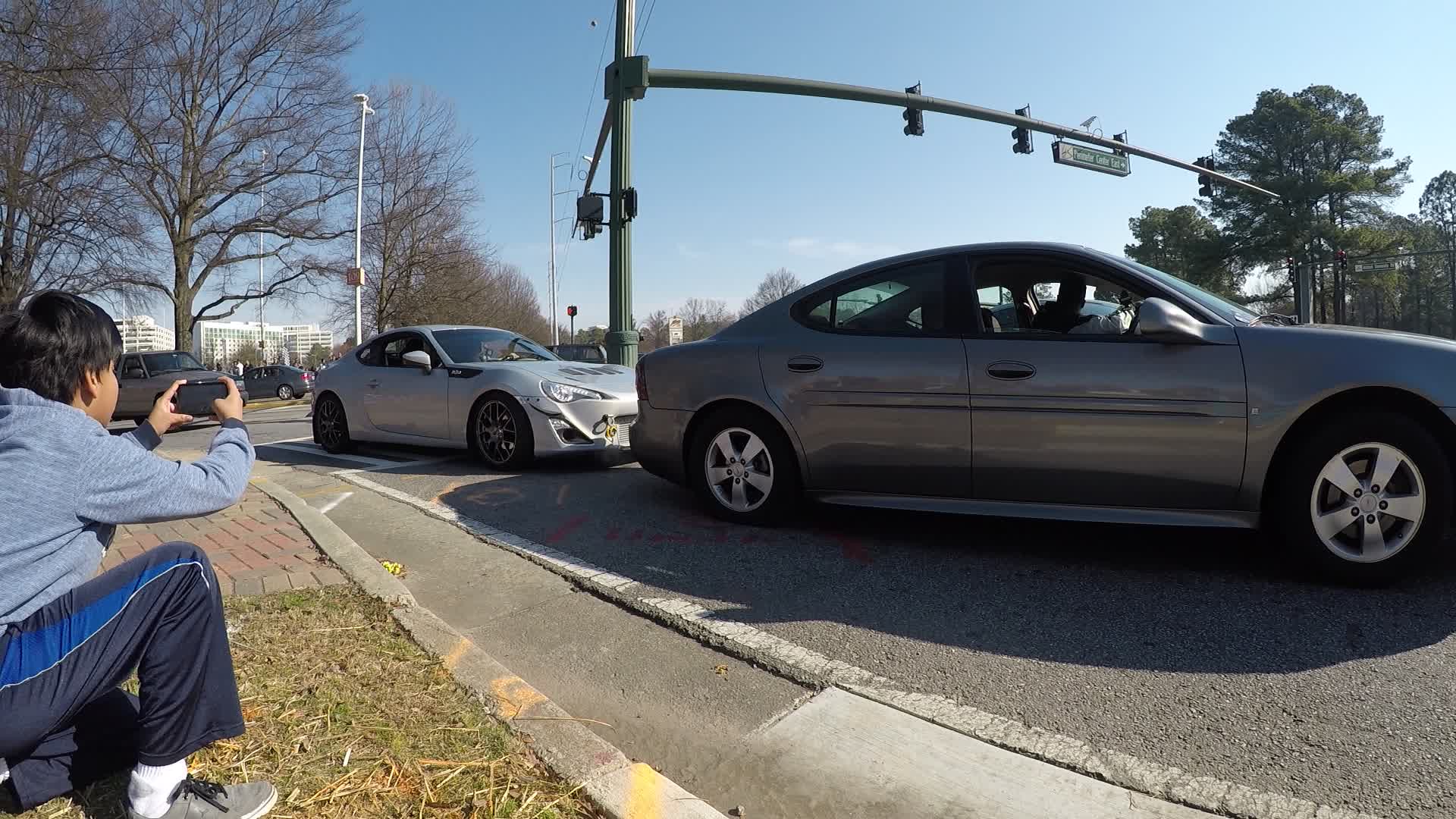The image shows two silver cars in motion, traveling along a road. The car in the foreground has black tires with silver rims and a driver inside who is glancing to the left. The vehicle itself has a grayish-silver hue. The second car, following closely behind, has darker rims and appears lower to the ground. This car too has a driver, who can be seen with a hand on the steering wheel.

In the background, there are various types of trees; some are evergreen pine trees while others are leafless, indicating a seasonal transition. The scene is set near a traffic light and a road sign that reads something like "Center's Exit."

On the left side of the image, a boy dressed in blue, with black hair, is visible. He is holding up a phone or camera, seemingly capturing the scene of the moving vehicles.